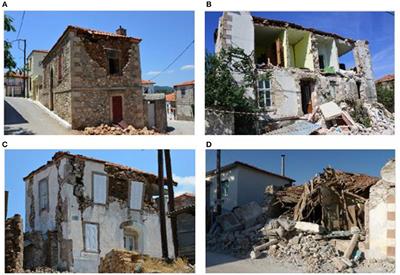This image is a composite split into four labeled sections: A, B, C, and D, each depicting the stages of a building crumbling. In the top left (A), there is a gray stone house with part of the second floor collapsed, with rubble blocking the front door. In the top right (B), a larger, four-bedroom house has its entire exterior wall crumbled onto the ground, accompanied by a tree in front. The bottom left (C) shows another box-like house with more windows, where the upper part has started to break off, scattering debris around. Finally, in the bottom right (D), the house is completely demolished, reduced to a pile of brick and some remnants of a red roof. Each photograph is set against a bright, blue daytime sky, suggesting outdoor scenes possibly hit by some calamity, giving a clear view of the gradual destruction leading to total ruin.